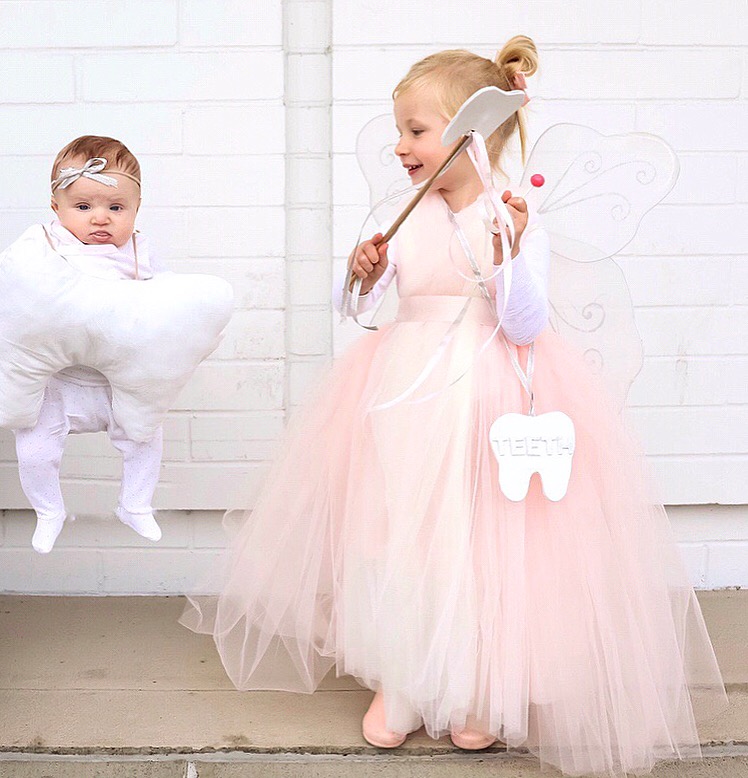The photograph features two children in costumes set against a white brick wall, standing on a beige concrete floor. On the right side of the image is a young girl, likely around three to five years old, dressed as a tooth fairy. She is adorned in a light pink, long-sleeved dress with a frilly skirt that extends to the floor, complemented by glittery transparent wings on her back. She has a ribbon tied around her torso, from which hangs a large white tooth-shaped medallion labeled "teeth." In her hand, she holds a wand topped with a matching tooth shape.

To the left of the girl is an infant, appearing to float in the air perhaps due to the way the photograph is framed. The baby, with short brown hair and a white bow on its head, is dressed predominantly in white pajama bottoms with dot patterns. The infant clutches a large white pillow resembling a tooth, contributing to an overall theme that suggests the baby is meant to represent a tooth, while the girl portrays the tooth fairy.